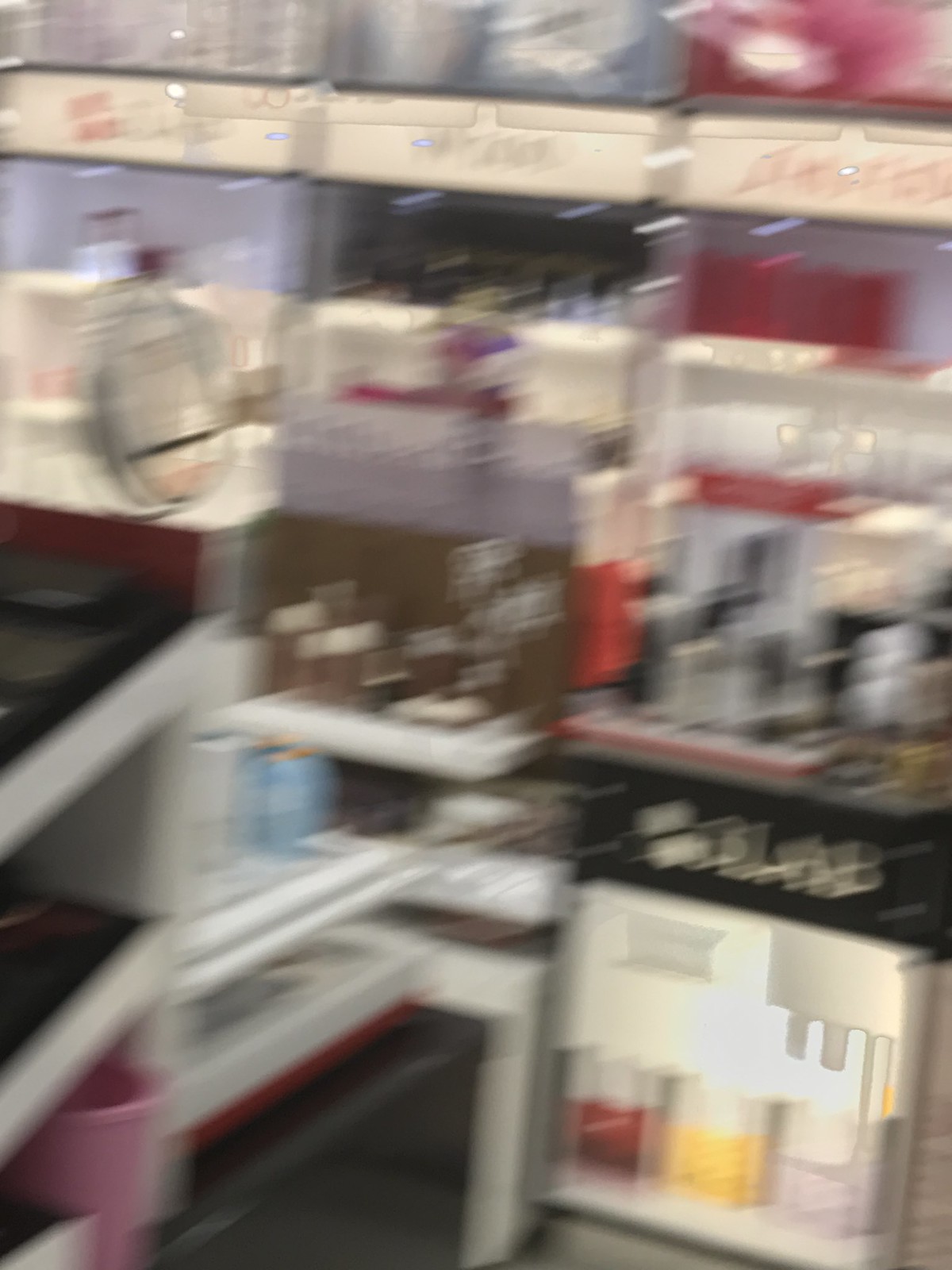A blurry photograph captures a beauty kiosk display at a shopping mall, characterized by its indistinct yet intriguing details. The image reveals an array of six display cases lined in a row, ascending toward the top of the photo. Amidst the blur, a small chair is discernible, likely intended for patrons to sit and have their makeup applied. Various bottles, possibly containing perfumes, are visible within the cases. Below this arrangement, another display case stands out with a sophisticated appearance, featuring a black header with what appears to be golden font, possibly forming the word "BLAB" or something similar. Tucked beneath are more bottles, perhaps additional perfumes, presented in an elegant manner. A round mirror is positioned to the left of the chair, adding a touch of functional beauty to the kiosk. Despite the lack of sharpness, the overall impression is that of a high-end perfume display within a mall setting.